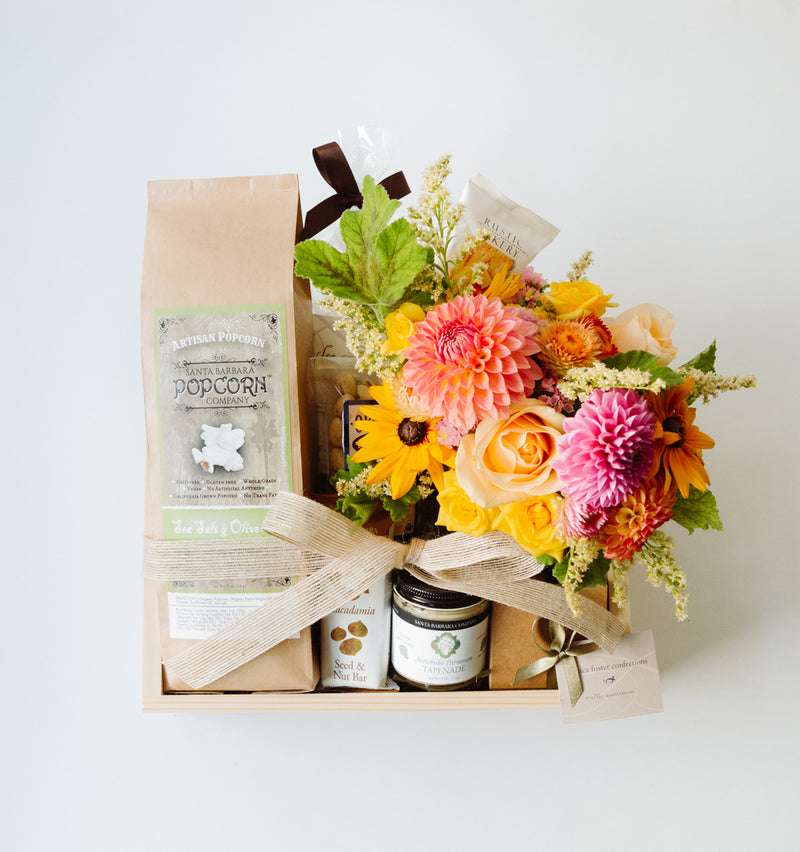This vibrant photograph captures an exquisitely wrapped gift basket arranged on an all-white background with soft gray shadows on the lower right side. The centerpiece is a light brown wooden box adorned with a cream-colored cloth bow that ties the entire presentation together. Inside, a tall brown bag of gourmet popcorn from the Santa Barbara Popcorn Company stands prominently on the left, boasting artisanal quality with sea salt and olive flavor. Flanking the right side of the box is a beautiful, lush bouquet featuring flowers in a kaleidoscope of colors: purple, pink, yellow, orange, red, and cream, accented with green leaves and a black bow on the top left corner.

Among the flowers, which include longer, yellowish-green stems, there’s also a smaller white bow adding an extra touch of elegance. Directly in front of the floral arrangement, an assortment of treats is neatly displayed: a white bag labeled "macadamia seed and nut bar" in two shades of brown lettering, and a mysterious jar that possibly contains jam or another delightful treat. To complete the ensemble, a small card sits in the bottom right corner next to a gold bow, all of which combine to create a luxurious and thoughtful gift, perfect for any celebration.